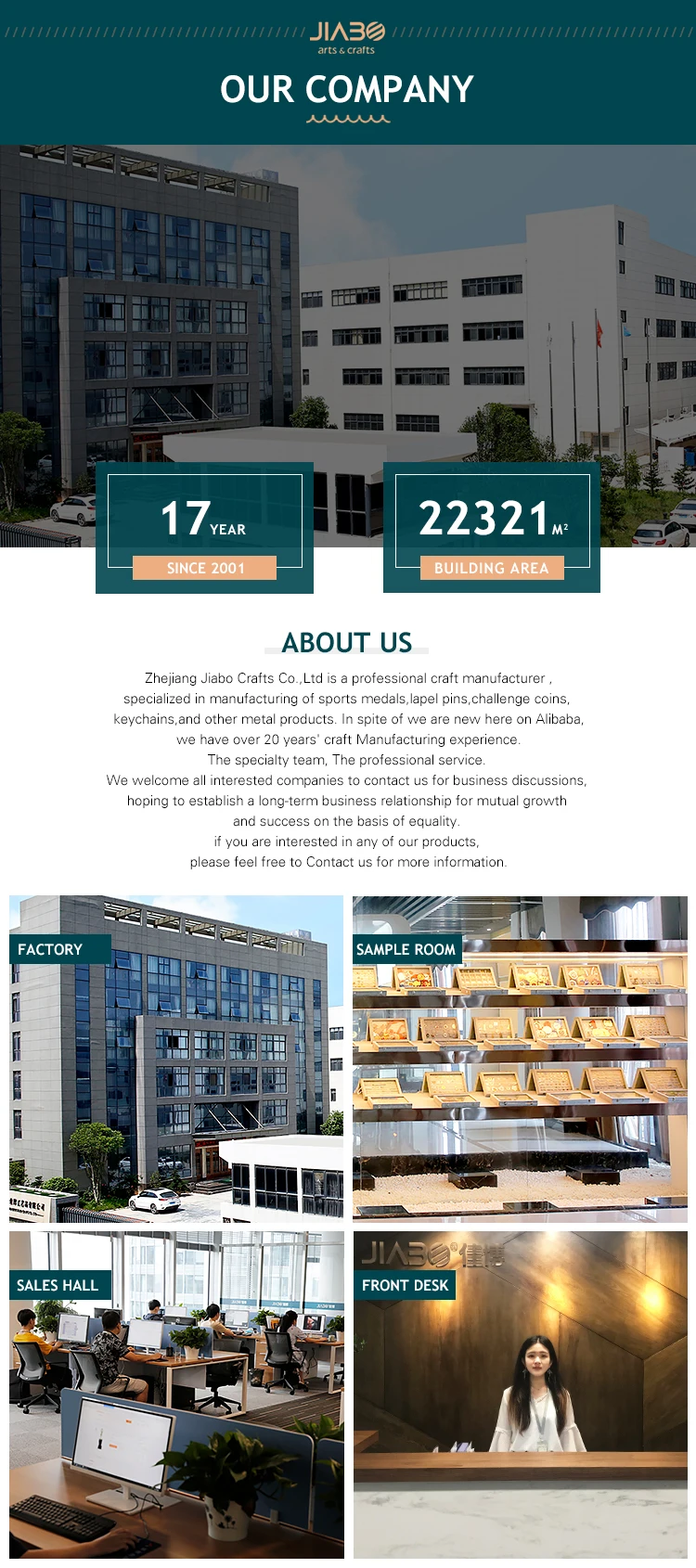This image is a detailed screenshot of a webpage or template from a company called Jibo. At the very top, the company's name, "Jibo," is prominently displayed. Below the company's name, there is large, bold text introducing the company. Further down, the image features a photograph of a substantial building adjacent to another structure, with cars parked alongside and a small grassy area with flags fluttering nearby.

The webpage contains two notable sections of text. One section highlights "17 years, since 2001," while the other provides details on the building's area and square footage. Centered beneath these sections is an "About Us" segment consisting of two paragraphs of small, hard-to-read text.

Directly below the "About Us" section are four distinct images. The first image showcases the primary building, identified as the factory. The second image depicts a sample room, providing a glimpse into the company's offerings. The third image shows the sales hall, where multiple individuals are seen working at their individual desks on computers. The fourth and final image features the front desk, where a woman is positioned behind the counter, welcoming visitors.

This structured layout offers an informative overview of Jibo's facilities and operations.